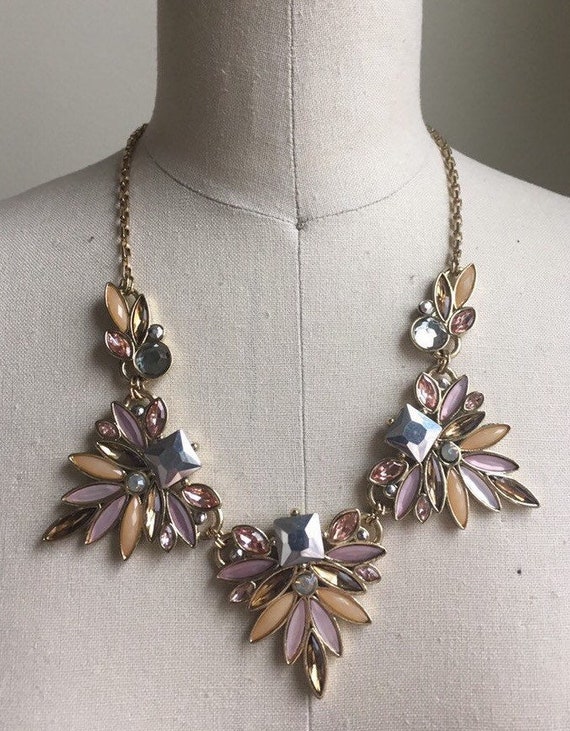The image depicts a fabric-like mannequin, light beige in color, set against a solid gray backdrop. The mannequin is shown from the neck down to just above the chest, showcasing an ornate necklace. The necklace features a gold chain adorned with detailed pendants. These pendants consist of a round jewel, an oval, and petal-shaped emblems, each embellished with colored gems in hues of light pink, light blue, and light orange. The design includes three identical, more elaborate segments alongside simpler decorative elements. This intricately designed piece of costume jewelry adds a touch of elegance to the mannequin's presentation.